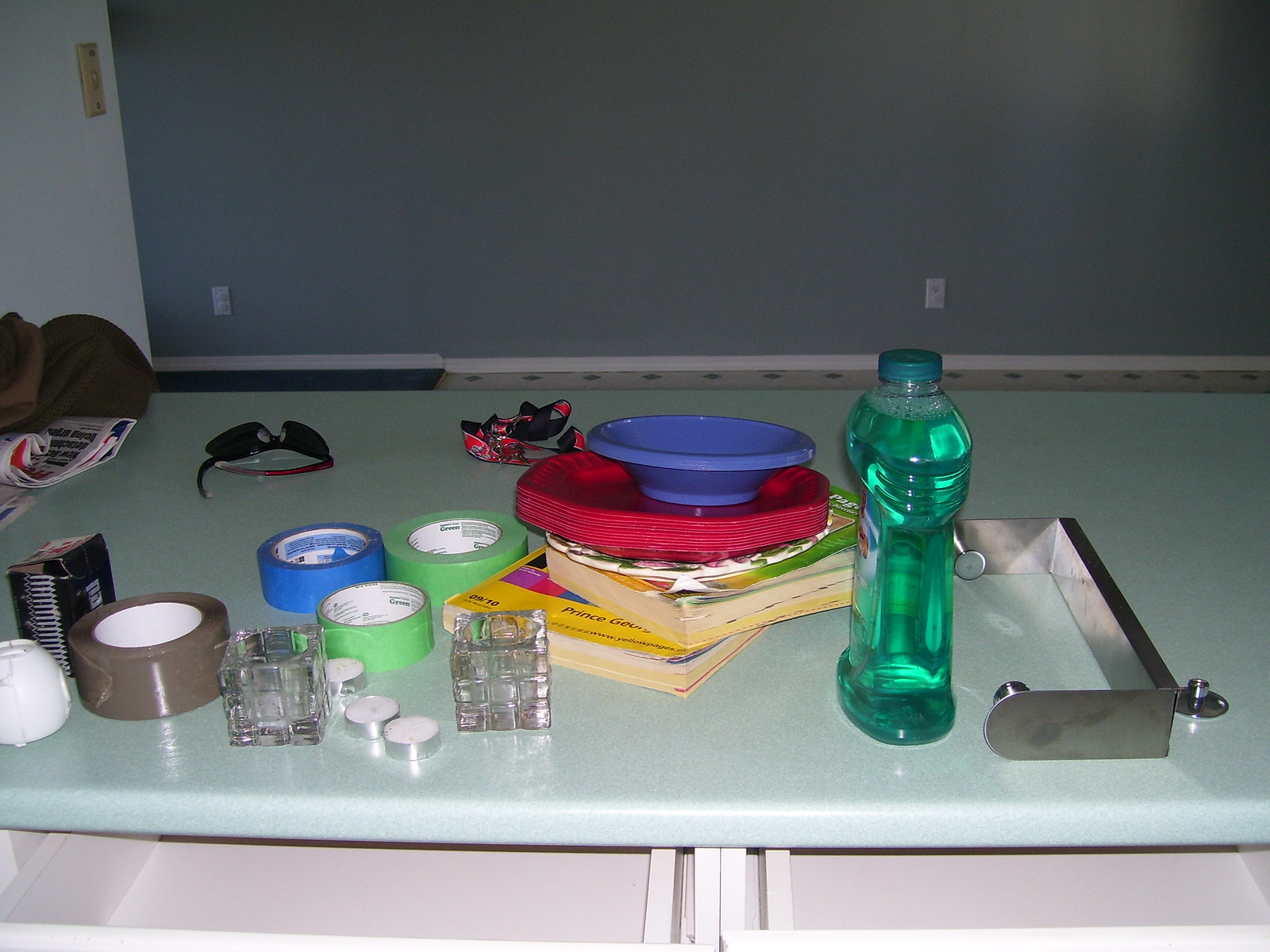The photograph presents a green table with several open drawers, positioned away from a grey wall. The floor, visible between the table and the wall, features homey tiling, suggesting a residential setting, potentially with small children given the presence of childproofing devices. The wall is equipped with a couple of electrical outlets with covers.

On the table's surface, a variety of items are scattered, giving it a bustling, lived-in appearance. Prominently displayed are four rolls of electrical tape in bright green, blue, and brown hues. Adjacent to these, two small, square candle holders approximately one to two inches wide are accompanied by three white tea lights.

To the left, there is a door handle safety device, presumably for childproofing. In the back left corner, rolled-up papers, possibly newspapers or mail, are slightly obscured by what might be a jacket or hat. Nearby, a pair of sunglasses and a lanyard, likely attached to a key, are also present.

Near the electrical tape, a stack of unidentified black items is visible. Towards the center of the table, two stacked books, resembling old-style phone books, are topped with a varied assortment of party plates—some red and hexagonal or octagonal, alongside smaller ones—and disposable blue bowls. 

On the right side of the table, a green bottle potentially containing soap or cleanser stands next to a detached silver chrome paper towel holder, adding to the utilitarian mix of items.